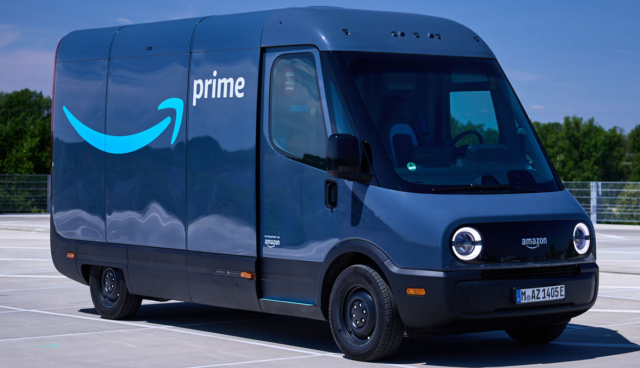In a bustling parking lot, clearly marked by white-painted lines delineating the parking spaces, an Amazon delivery van commands attention in the foreground. The setting is framed by a backdrop of a chain-link fence, intertwined with patches of a see-through material, allowing glimpses of verdant, green trees. Above, the sky stretches in a perfect, uninterrupted blue, suggesting a bright, clear day.

The focal point of the image, the Amazon van, is a deep, dark blue, with a distinctive light gray and bluish pattern along its lower edge, reminiscent of soft, wispy clouds. Adorning the side of the van is Amazon's emblematic turquoise arrow, elegantly curved to resemble a smile, hinting at the convenience and service the brand promises. Below the arrow, the word "Prime" is prominently displayed.

The van is equipped with a long, European-style license plate on its front, featuring a blue vertical strip on one end, contrasting against the dominant white background, with a series of bold black letters and numbers. Practicality is evident with the presence of a sliding door on the side, designed for efficient delivery service. The vehicle rests on sturdy black tires, ready for its next journey.